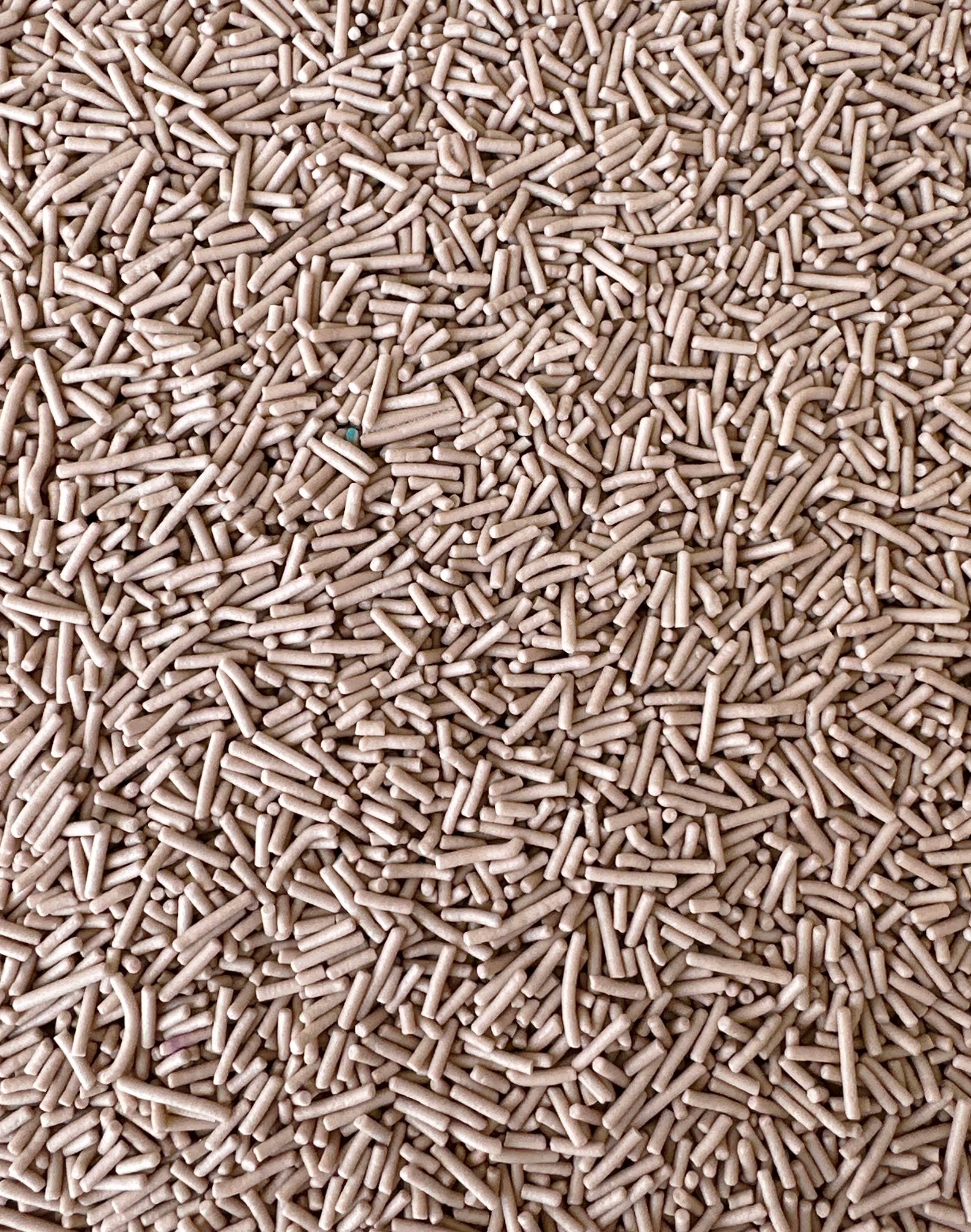This macro photograph showcases a densely packed pile of long, cylindrical objects, creating an intricate pattern that fills the entire frame. These objects, of varying sizes but predominantly similar in appearance, feature a predominantly gray-brown color with hues of green, purple, black, white, yellow, and tan interspersed throughout. Amidst this sea of tiny pieces, there is a notable bluish object—possibly the head of a nail—located about a third of the way down the left corner, adding a touch of mystery. The texture of these cylinders is ambiguous, suggesting they could be made of plastic or metal. Despite some visual resemblance to cut spaghetti or even sprinkles used on desserts, their true nature remains indistinct, adding to the enigmatic quality of the image.